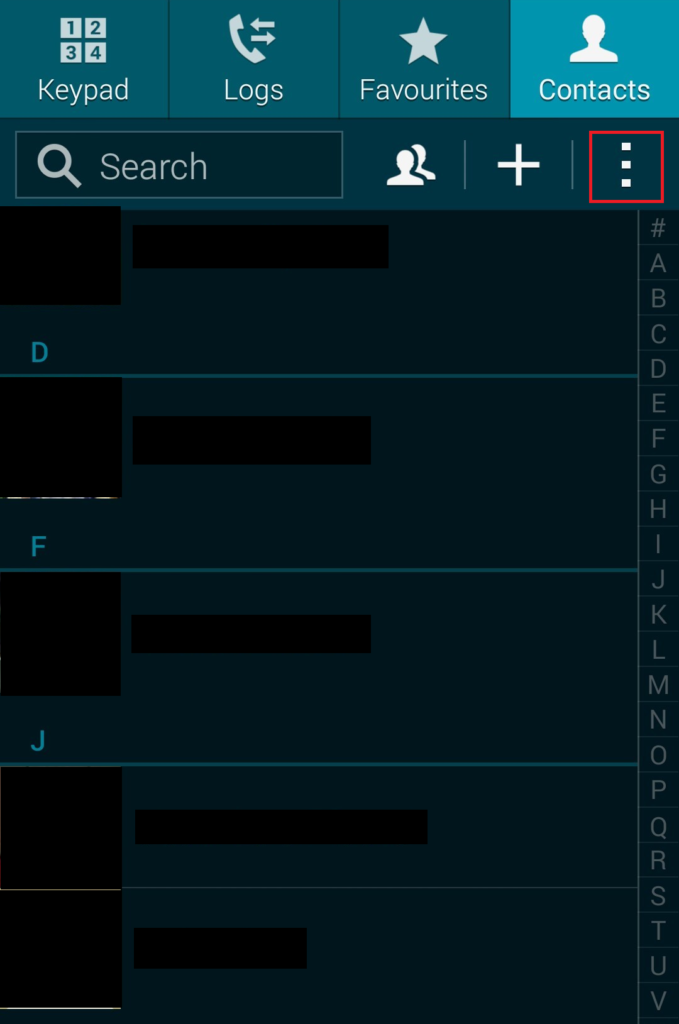This image appears to be a screenshot of a digital interface, likely from a mobile device or software application. The screenshot is from an unidentified source and contains several blacked-out sections. At the top, there are four squares arranged in a grid labeled "one," "two," "three," and "four," with a header denoted as "Keypad."

Directly below this grid, there are icons and labels indicating different functionalities:
- An icon of a phone handset labeled "Logs."
- An icon of a star labeled "Favourites" (notably spelled with a 'u' in the British manner).
- An outline of a person labeled "Contacts."

Beneath this section is a search bar, presumably for searching contacts or entries within the application.

To the left of the search bar is an icon featuring two silhouettes with a white plus sign, indicating the option to add new contacts or entries.

Next, there are three vertically aligned squares, which are highlighted in red, drawing particular attention within the interface.

Below the highlighted area, there are several rows with labels such as "D," "F," and "J." This section includes the areas that have been redacted or blacked out.

On the far right side of the image, there is a vertical alphabet starting with a number sign (#) and continuing up to the letter "V," though it is cut off at the bottom of the screenshot.

The orientation of the image is portrait, indicating it is taller than it is wide. The screenshot notably lacks any living entities or vehicles:
- No people, animals, birds, plants, flowers, or trees.
- No automobiles, airplanes, or helicopters.

This description highlights the methodical and structured layout of the interface captured in the screenshot.